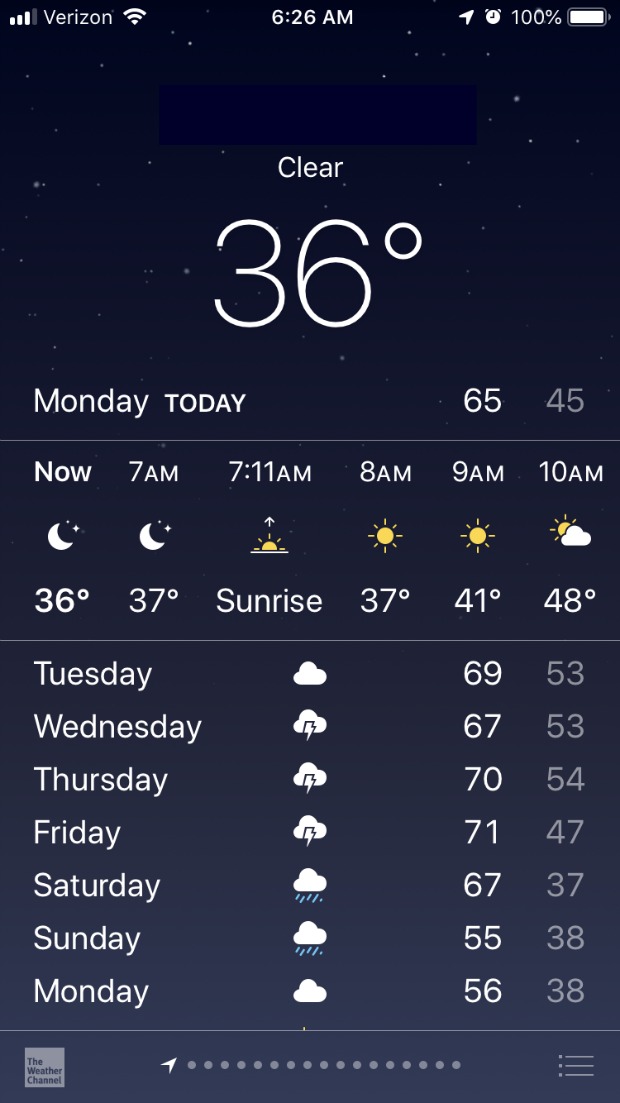This image captures a smartphone displaying a weather app with detailed forecasts. The screen shows the current temperature is 36°F with clear skies, as indicated by a starry, dark background—suggesting it is still early morning before sunrise. The time on the phone reads 6:26 a.m., and the app indicates that the temperature will increase slightly to 37°F by 7 a.m. and remain the same until 8 a.m. The sun is expected to rise at 7:11 a.m. As the morning progresses, the temperature will reach 41°F by 9 a.m. and 48°F with partly cloudy conditions by 10 a.m. 

The weekly forecast starts with Monday, which has a high of 65°F and a low of 45°F. The weather for the following days is as follows:
- **Tuesday:** Cloudy with a high of 69°F and a low of 53°F.
- **Wednesday:** Rainy with thunderstorms, a high of 67°F, and a low of 53°F.
- **Thursday:** Rainy with thunderstorms, a high of 70°F, and a low of 54°F.
- **Friday:** Rainy with thunderstorms, a high of 71°F, and a low of 47°F.
- **Saturday:** Rainy, a high of 67°F, and a low of 37°F.
- **Sunday:** Rainy, a high of 55°F, and a low of 38°F.
- **Next Monday:** Cloudy with a high of 56°F and a low of 38°F.

The app differentiates the type of rain across the week: Wednesday, Thursday, and Friday feature rain showers accompanied by lightning bolts, while Saturday and Sunday display blue rain clouds, indicating simpler, sustained rain. This degree of specificity helps in preparing for the week's varied weather conditions.